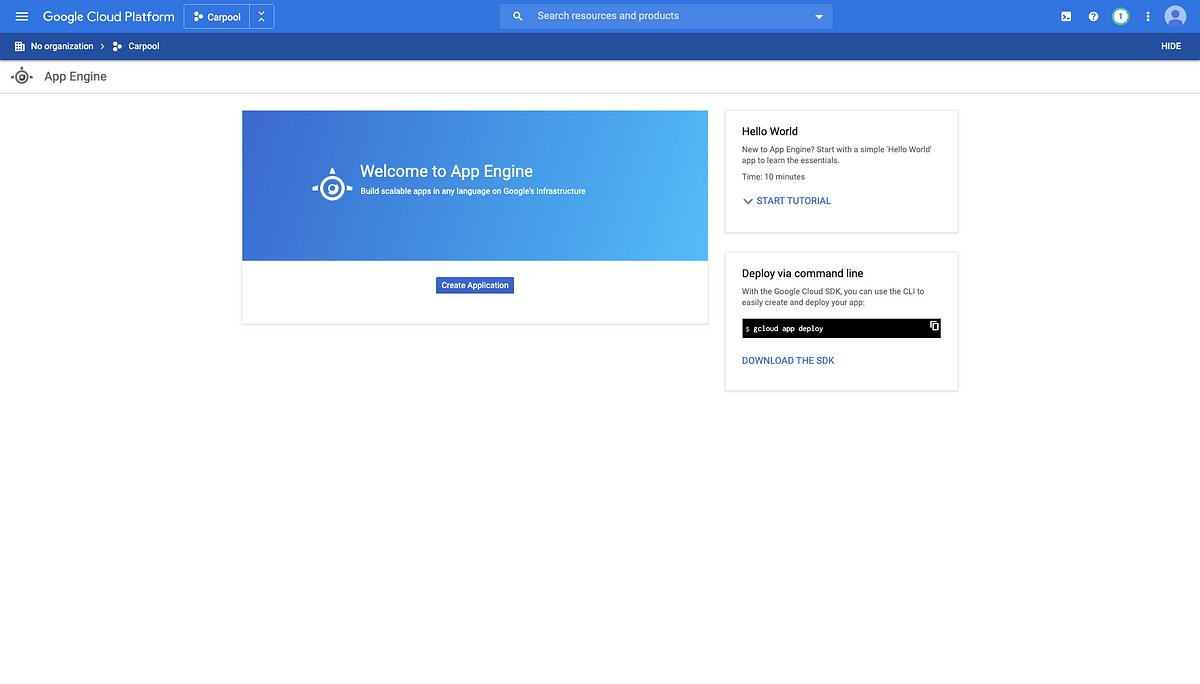This is a detailed and cleaned-up caption describing a cropped screenshot of the Google Cloud Platform homepage:

The image represents a cropped screenshot of the Google Cloud Platform homepage. The header at the top left prominently displays "Google Cloud Platform". Centrally located is a search bar. In the far right corner, there is a generic user profile icon set against a blue background, blending subtly with the page.

Dominating the right center of the page is a large rectangular image welcoming users to App Engine, accompanied by a line of white text underneath. To the left, towards the top, there is a small box labeled "Hello, world", introducing itself. Directly below this, a white box contains the text "display via command line", followed by a dropdown menu. 

The rest of the page is largely blank. Below the header bar on the top left, the word "App Engine" is displayed with a small corresponding logo to its left.